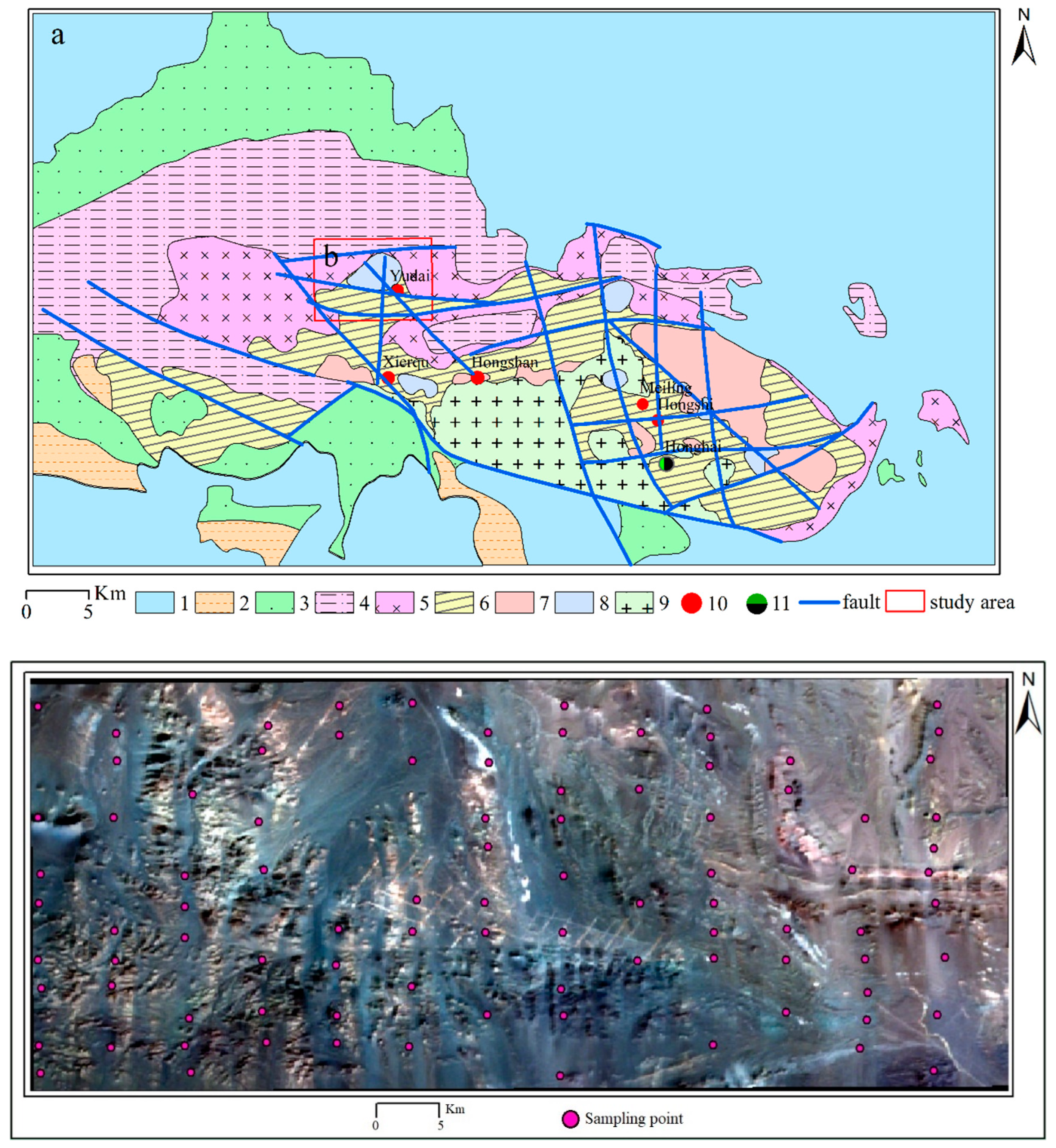The image is a composite of two separate images stacked vertically. The top half is a meticulously drawn, rectangular map framed by a thin black border with a white inner margin, and a second thin black line. This map features a varied palette of colors including greens, pinks, yellows, oranges, reds, and blacks, all corresponding to geological or geographical features explained in an accompanying legend located below. The background of the map is blue, and the land structure is outlined in black. Several areas are marked with red dots and labeled with black text reading "Yu Dai," "Zerkyu," "Hongsman," "Meiling," "Hongyu," and "Hongkai." The upper left-hand corner of this image includes the letter "A," and the right-hand corner features an "N" with an arrowhead pointing north. Additionally, there are blue lines on the map indicating faults, and a red box labeled as the study area marked "B."

The bottom half contrasts sharply with the top, offering a more realistic satellite photograph with a predominantly pink and dark blue coloration which represents various types of land cover or areas. This image is also rectangular and contains multiple pink dots denoted as "sampling points" in the legend. The scale for this part of the image is provided, measuring distances from zero to five kilometers. Together, these two images provide a detailed representation combining both artistic and realistic elements to convey geological and geographical information.